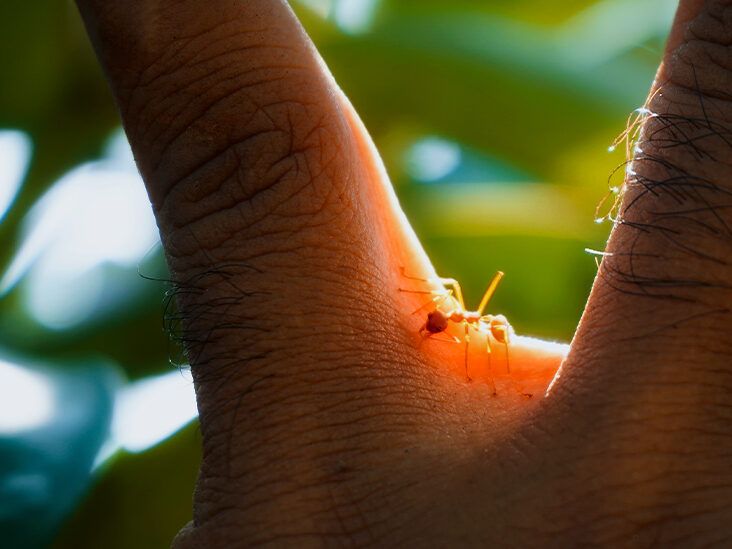This vividly detailed, close-up photograph captures two fingers of a presumably older man, separated in a V-angle, taking up the whole center of the image. The fingers, adorned with black hair near the knuckles and marked with wrinkles, suggest the hand of a mature individual. Nestled in the web space between the fingers, highlighted by the reflecting sunlight on a bright, sunny day, is an ant. The photograph reveals intricate details of the ant, including its head, body, legs, and even its jaws, emphasizing the high level of zoom. The background is out of focus but hints at a lush, green environment, possibly a park, adding a natural and serene backdrop to the contemporary, realistic photograph.